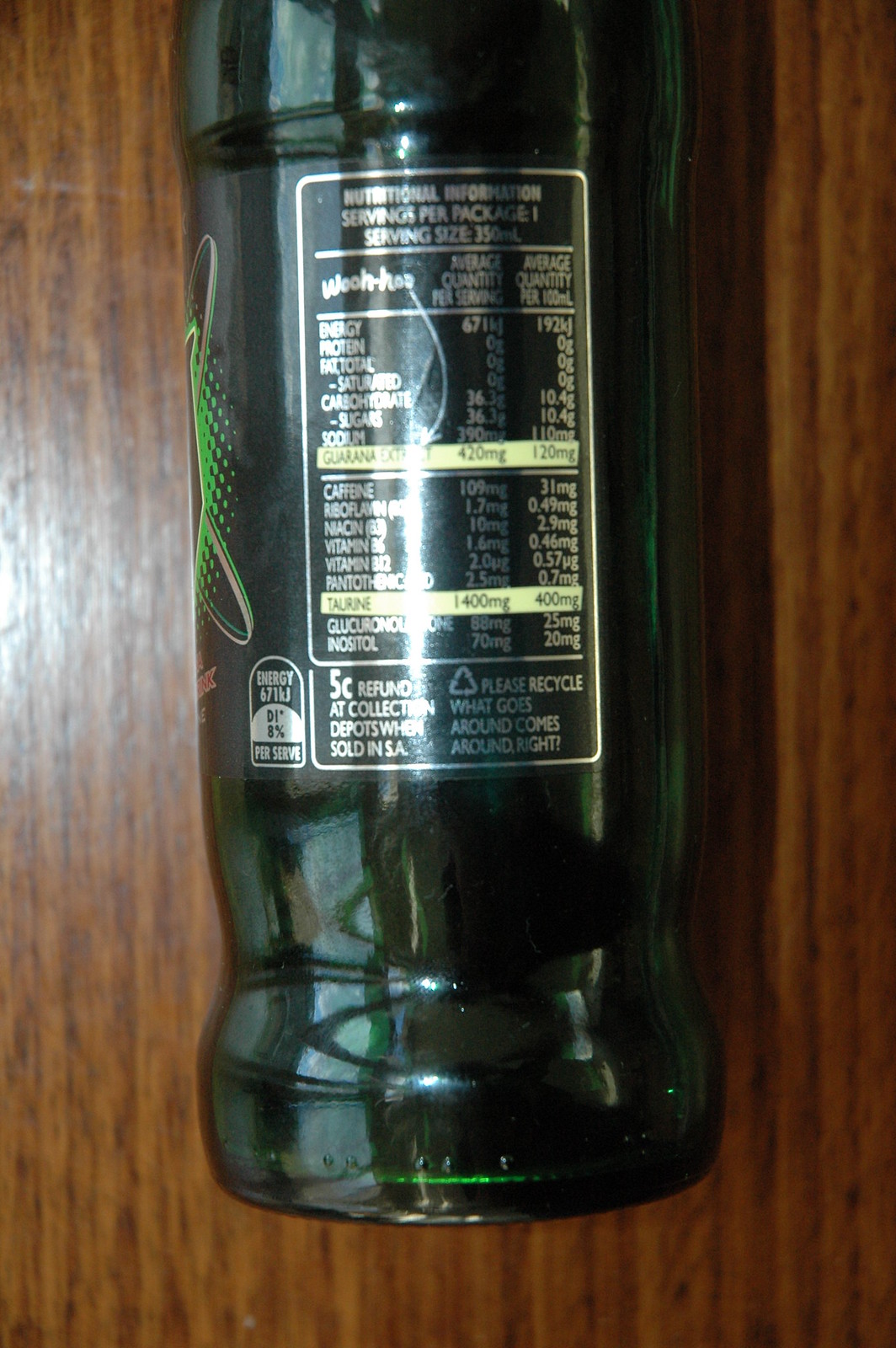The image features a close-up of a black bottle, likely an energy drink, lying sideways on a dark brown wooden table with grains running vertically. The bottle has a green design on the label, and no brand name is visible. The prominent nutritional label lists various ingredients including caffeine, riboflavin, niacin, vitamins B6 and B12, glucuronolactone, and inositol, with a serving size of 350 milliliters. The label includes instructions to recycle with the phrase "what goes around comes around," and mentions a 5 cent refund at collection depots when sold in SA. The energy content is specified as 671 KJ per serve, and the photo is taken in portrait mode, capturing three-quarters of the bottle.